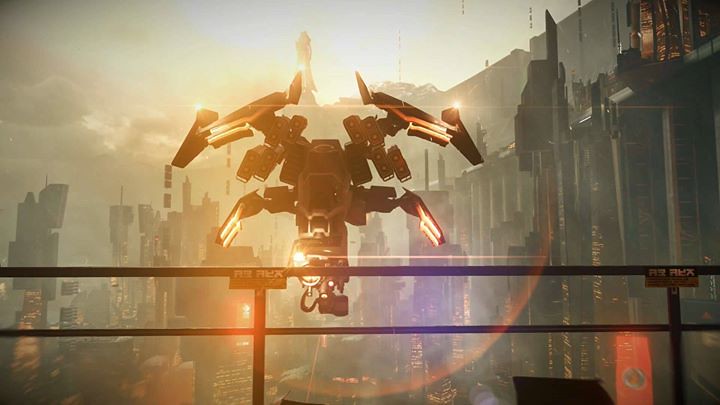The image depicts a dystopian, sci-fi cityscape under a dramatic sky, where the left side has a greenish-pink hue transitioning to a blue-green tint on the right. In the center and extending to the right are various buildings, partially obscured by intense sunlight and cloud cover. A prominent feature is a mechanical, robot-like figure with a red glow. This figure, which resembles a transformer, has extended arms and legs, and mechanical wings emanating light. It stands behind a black fence, which has signs with unreadable text. To the lower right, behind the fence, there is a red rectangle with a tan circle. The whole scene has a mix of colors, with the sky and sunlight creating dramatic visual effects and casting a dystopian feel over the entire cityscape.